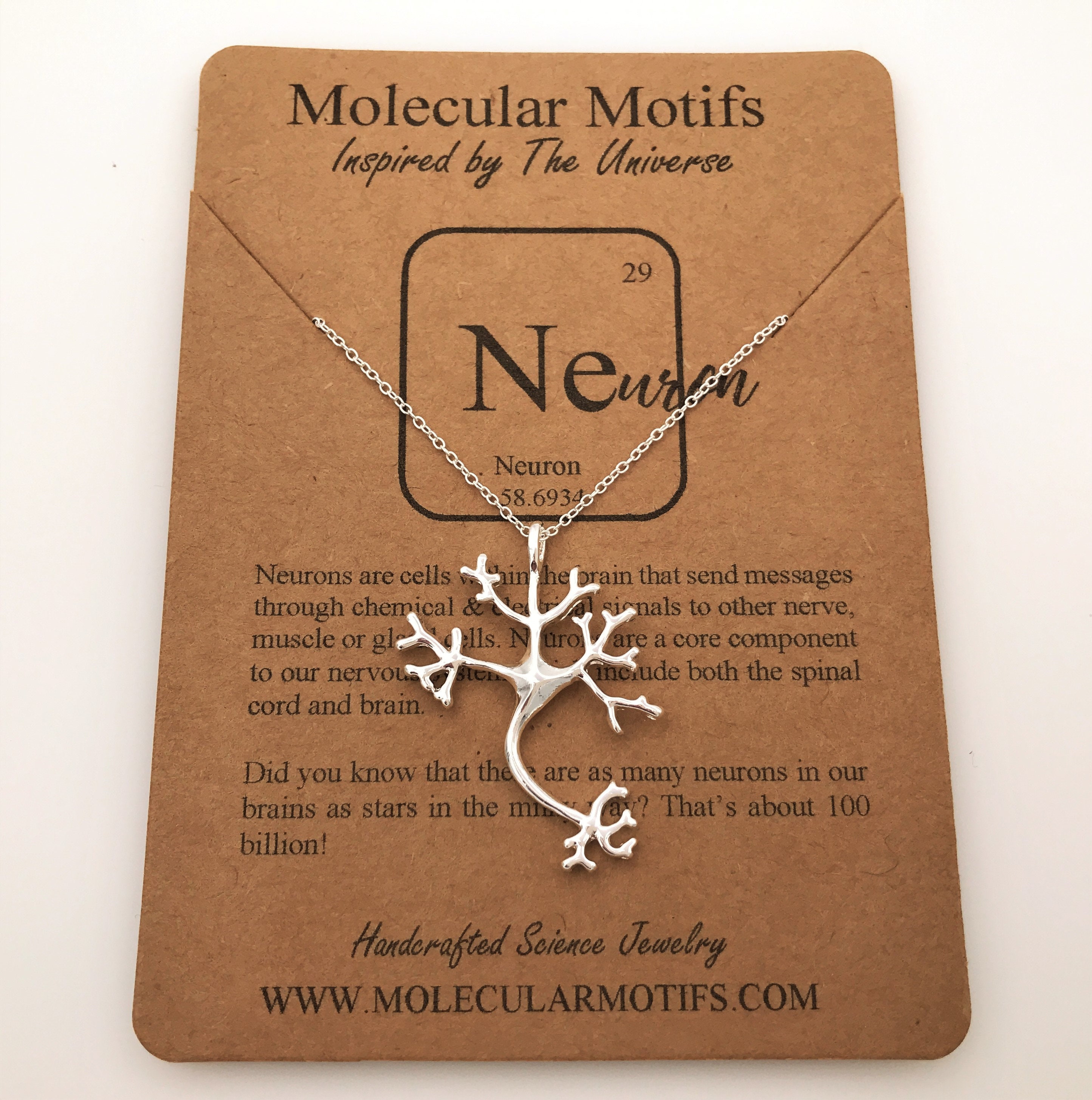The image showcases a piece of finely crafted jewelry prominently displayed against a brown card. At the front and center, the brown card features an exquisite silver necklace. The necklace consists of a delicate silver chain and a captivating pendant that resembles interconnected tree branches, evoking a sense of natural elegance and complexity.

At the top of the card, the text reads, "Molecular Motives - Inspired by the Universe. N.E. 29 Neuron 58.6934." Below the necklace, a detailed inscription elaborates on the significance of neurons: "Neurons are cells within the brain that send messages through chemicals and signals to other nerve, muscle, or cells. Neurons are a core component of our nervous system that includes both the spinal cord and the brain. Did you know that there are as many neurons in our brains as stars in the Milky Way? That's about 100 billion."

The bottom of the card provides a final touch, pointing to the origin of this unique item: "Handcrafted Science Jewelry - www.molecularmotives.com."